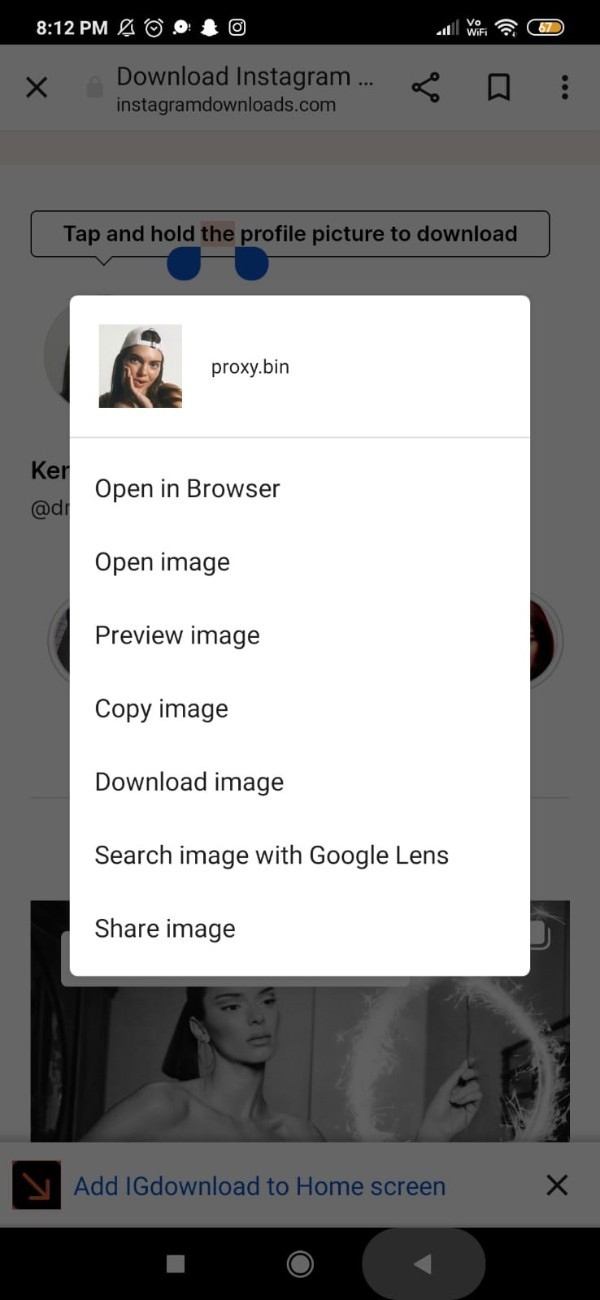A detailed screenshot taken on a smartphone at 8:12 PM shows a grayed-out screen with an active pop-up overlay. The smartphone has a 67% battery level, Wi-Fi enabled, and 3 out of 5 signal bars. The status bar displays the Snapchat and Instagram icons, with no new notifications or alarm set.

The background screen depicts a webpage from “instagramdownloads.com” with options to share, bookmark, close, and access a three-dot menu. The text instructs users to "tap and hold the profile picture to download," highlighting the word "the" with two blue teardrop markers indicating text selection.

At the screen's bottom, there's a brown square with a yellow downward-right pointing arrow, suggesting users can "add IG download to home screen." It shows regular Chrome browser buttons at the bottom.

The pop-up overlay, occupying about 80-85% of the screen, features a white rectangle with a photo of Kylie Jenner. In the image, she supports her chin with her right hand while wearing a backward-turned mesh baseball cap. Next to her picture, the text reads "proxy.bin" with a thin yellow line extending across the width below the image. Below, a list of seven clickable options includes: "Open in browser," "Open image," "Preview image," "Copy image," "Download image," "Search image with Google Lens," and "Share image."

Additional, indistinguishable text and images are visible behind Kylie Jenner's photo, including another image of her holding a sparkler at the bottom of the screen.